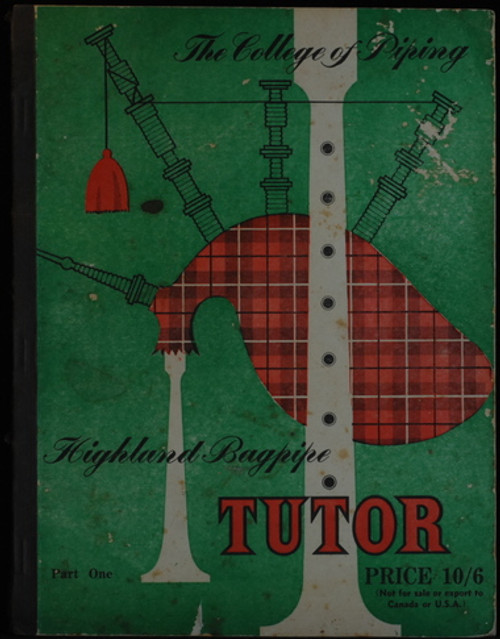The image, likely a book cover or a poster, features an illustrated Highland bagpipe adorned with traditional Scottish colors: red, black, and white in a crisscross plaid design. At the top, the text "The College of Piping" is prominently displayed, followed by a horizontal line. Below this line, the bagpipe illustration occupies the central space with its bag displaying the typical plaid pattern. To the left of the bagpipe, the text "Highland Bagpipe" appears in cursive. Superimposed over the bagpipe, there is a white wind instrument resembling a flute with seven holes arranged vertically. Beneath "Highland Bagpipe," bold red letters outlined in black spell out "Tutor." Further down, additional text states "Price 10/6" and "Part 1," with the note "Not for Sale or Export to Canada or USA" located underneath the price. The overall style is detailed and illustrative, blending elements of both a product advertisement and a traditional educational publication.